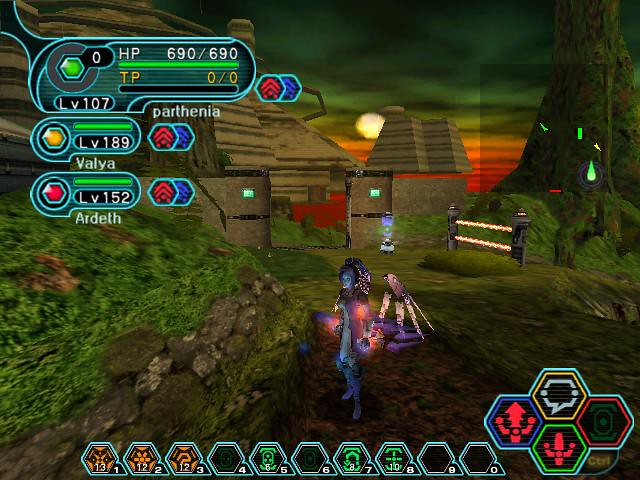The screenshot depicts an engaging scene from a 64-bit video game, characterized by its polygonal graphics. In the upper left corner of the image, three rounded rectangles display crucial information about the player's characters. The top rectangle shows "HP 690 / 690," indicating the player's health status is at its maximum. Below it, details for three characters are listed: Valya at level 189, Ardith at level 152, and Parthenia at level 107.

The bottom section of the screen features a row of ten hexagons. Four of these hexagons are blank, while the remaining six are split between green and orange symbols, three of each color. In the bottom right-hand corner, another set of four hexagons is present, each adorned with symbols correlating to different in-game functions or abilities.